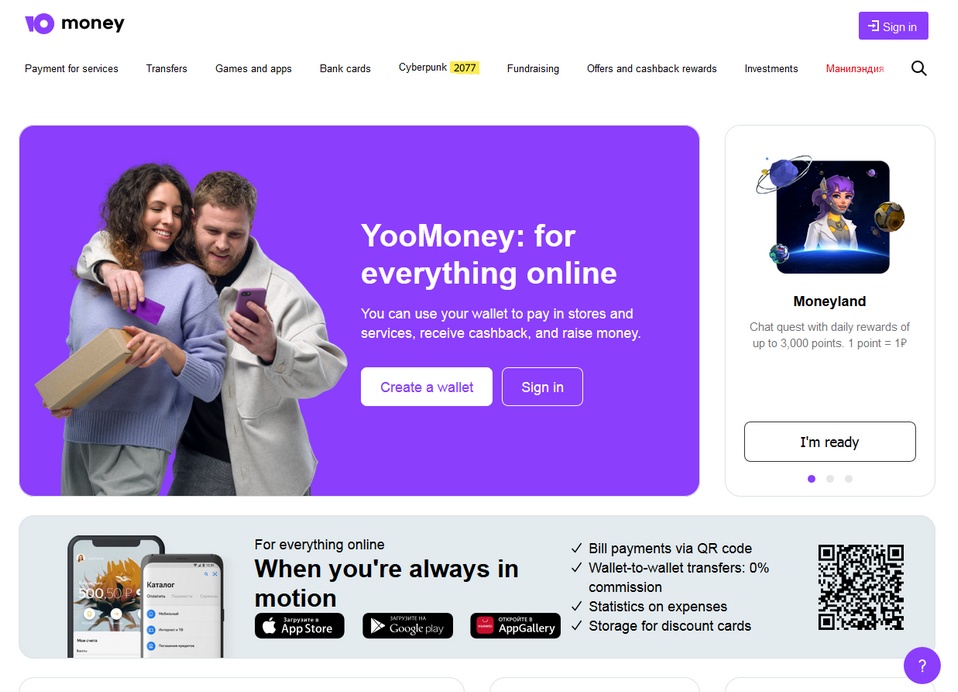Here is a detailed and cleaned-up caption for the image described:

---

This image is a detailed screenshot of the YouMoney (spelled Y-O-O-M-O-N-E-Y, all one word) website. The upper-left corner prominently features the company logo, which consists of a purple circle with a white dot in the center, accompanied by a short line to the left, and the word "money" written in lowercase black font. The background is white, providing a clean contrast.

Below the logo, a menu lists various options: "Payment for Services," "Transfers," "Games and Apps," "Bank Cards," "Cyberpunk 2077," "Fundraising," "Offers and Cash Back Rewards," and "Investments." Additionally, there's a word in a foreign language written in red font.

Centered on the page is a purple rectangle featuring the company name "YouMoney" in bold white font, followed by a colon and the tagline "for everything online." Beneath this tagline, more text in white (but not bold) reads, "You can use your wallet to pay in stores and services, receive cash back and raise money."

To the left of this text, there is an image of two people against a purple background (the original photo’s background has been removed). The image shows a white man and woman looking at a smartphone he is holding. The man, who has brown hair, a beard, and a mustache, is wearing a white shirt and has his arm around the woman's right shoulder. The woman, also with brown hair, is clad in a light blue sweater.

Directly beneath this section is a light blue banner with the headline, "When you're always in motion." This banner also displays icons for the App Store (iPhone), Google Play, and the Samsung App Gallery, signifying available downloads for the YouMoney app. In the lower right corner, there is a QR code accompanied by a list of features: "Bill Payments via QR Code," "Wallet to Wallet Transfers," "0% Commission," "Statistics on Expenses," and "Storage for Discount Cards."

---